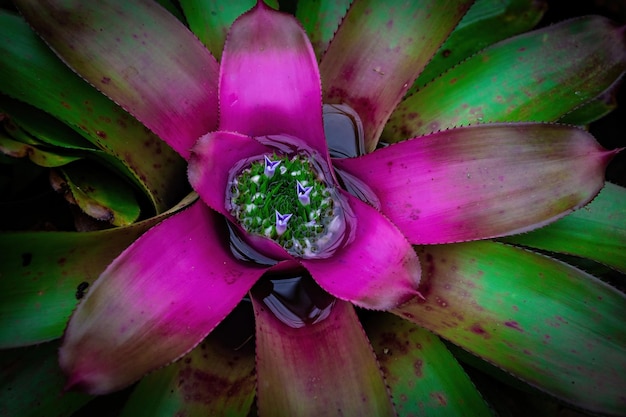This painting presents a mesmerizing view from above, capturing the intricate interior of a plant or flower with remarkable detail. Surrounding the scene is a cluster of lengthy, oblong leaves, characterized by their serrated edges. These leaves transition in color from rich purples at the core to vibrant greens with purple speckles on the lower layers, giving them a sharp and potentially cutting appearance. The waxy texture of the green leaves suggests resilience to rainy environments. The centerpiece of the artwork is striking, featuring an almost surreal vignette. Here, instead of the usual seed pod, viewers can see an image resembling a field of grass, adorned with three small purplish objects and additional white elements scattered within the greenery. This imaginative artistic choice adds a unique layer of depth, framing what appears to be a miniature landscape within the flower’s heart. The purple leaves, resembling petals, extend outward in various directions, creating a crown-like structure that enhances the overall composition's visual intrigue.